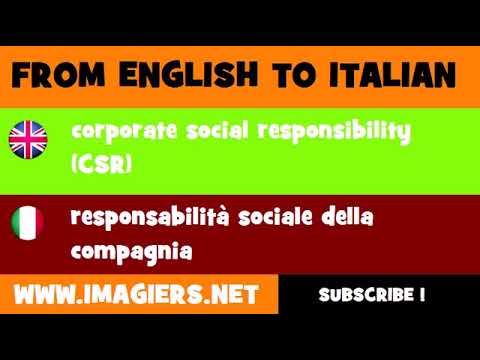The rectangular image is slightly wider than it is tall, framed by black horizontal rectangles at the top and bottom. It appears to be a digital advertisement containing a series of colored rectangles stacked vertically. At the top, in an orange rectangle, black text in all capital letters reads, "FROM ENGLISH TO ITALIAN." Below this is a neon green rectangle featuring a spherical British flag on the left and white, lowercase text that reads, "Corporate Social Responsibility," followed by "CSR" in all capital letters within parentheses. Directly beneath, a dark red rectangle displays a circular Italian flag on the left and lowercase text that states, "Responsabilità Sociale della Compagnia." Towards the bottom of the image, a yellow rectangle includes the website "www.imagineers.net" in white capital letters, and adjacent to it, in a black rectangle, is the word "SUBSCRIBE" in white capital letters with an exclamation point.